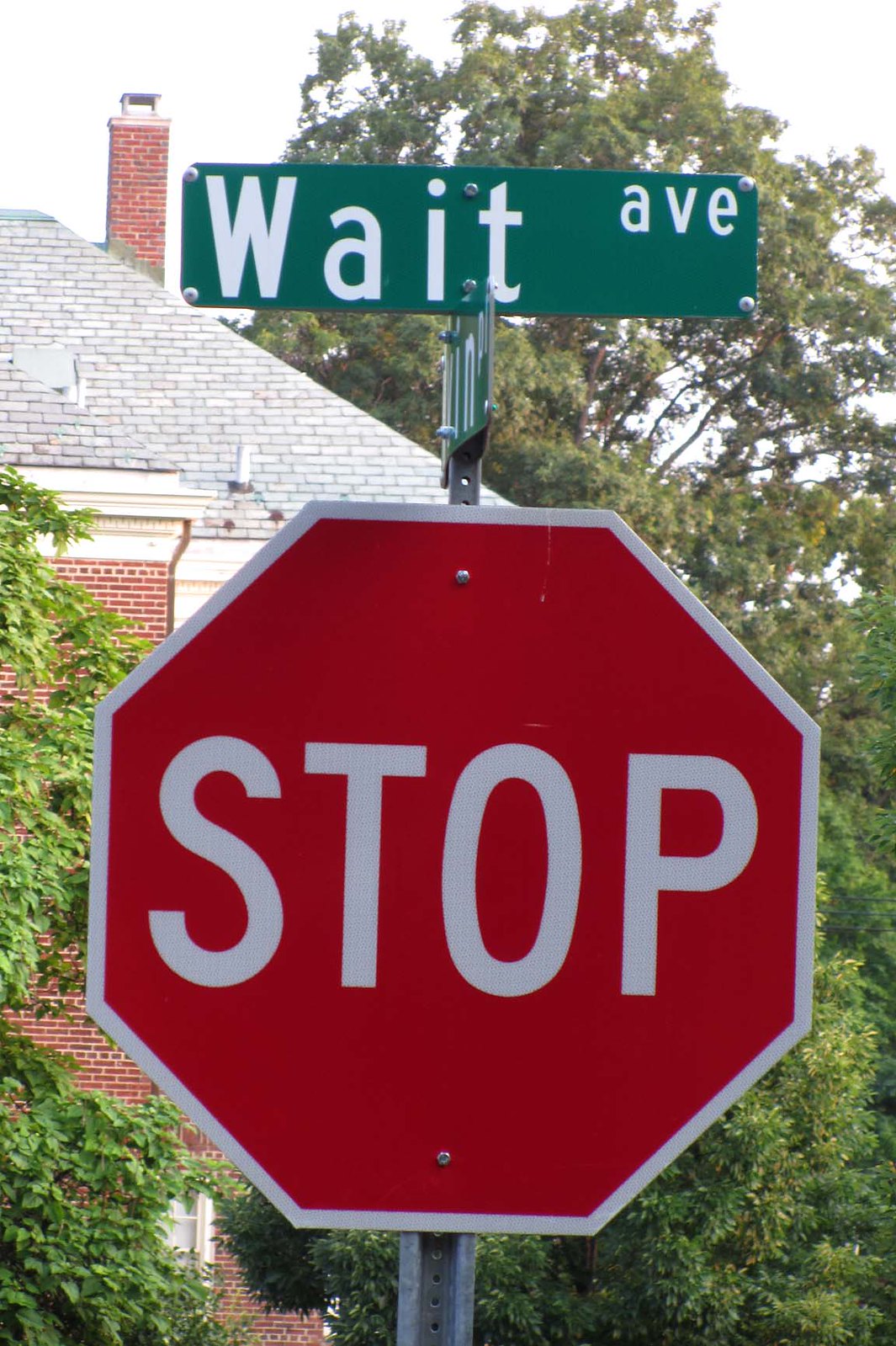In this picturesque scene, a cluster of street signs takes center stage amidst a lush, green backdrop. Dominating the image is a classic octagonal red stop sign, outlined in white with the word "STOP" boldly emblazoned across it. Above, a green street name sign reads "Wait Avenue," cleverly aligning to suggest "Stop and Wait."

To the right, a charming red brick building with a sloped gray shingled roof adds architectural interest. A red brick chimney punctuates the roofline, rising into an overcast yet bright sky that casts a diffused light over the scene. Verdant trees frame the composition on both sides, their leaves providing a natural contrast to the man-made elements. In the bottom right corner, a glimpse through the foliage reveals a window in the brick building, adding a subtle layer of depth and intrigue.